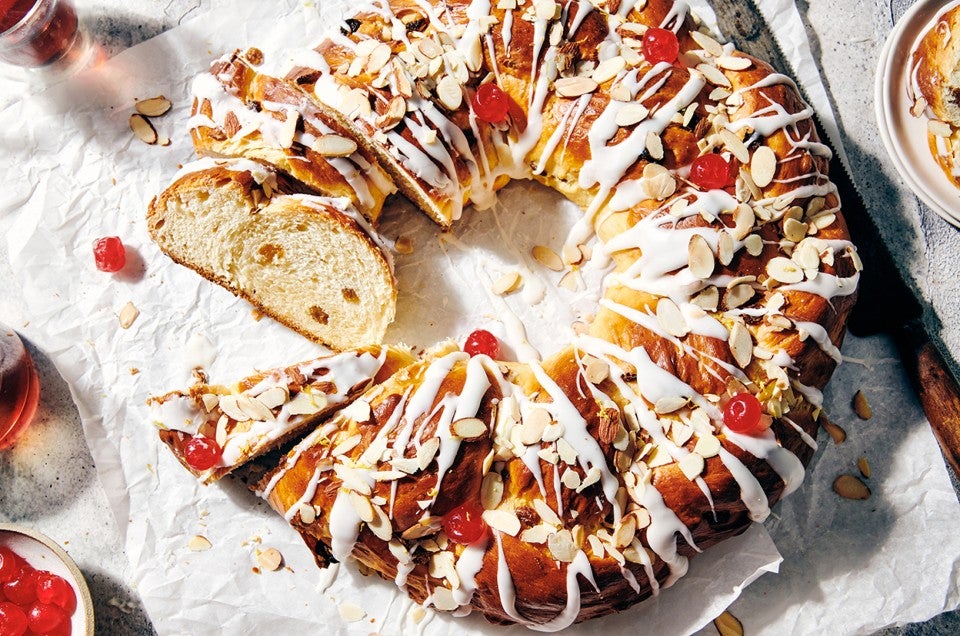This color photograph, taken from above, showcases a round, ring-shaped pastry with a hole in the middle, resembling a braided Christmas bread. The pastry, sitting on a white parchment paper atop a gray granite countertop, features a rich brown crust. The bread is adorned with whole candied cherries, raisins, and sliced almonds, all drizzled with thick, streaky white icing. The interior reveals a mix of candied fruits, including red and orange pieces that suggest apricots, cherries, and possibly pineapple, embedded within the dough. Beside the bread, a slice has been cut, showcasing its fruit-filled interior. Accompanying the pastry, on the left side of the image, are a bowl containing more candied cherries, a clear glass with an amber liquid, and some almond shavings scattered around. A knife lays nearby on the white tablecloth. This detailed depiction captures the festive, indulgent nature of this holiday treat.